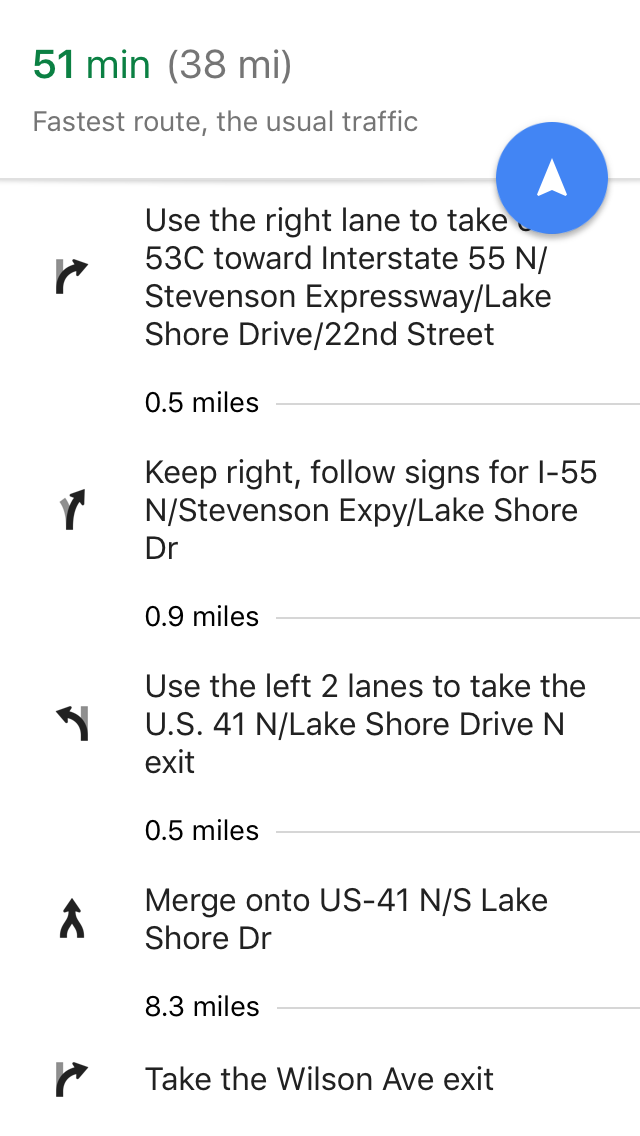The image shows a set of GPS directions to a searched location, emphasizing detailed navigational instructions. At the top, the display indicates a duration of 51 minutes with a distance of 38 miles, labeled as the fastest route with usual traffic conditions. Below this, there are five specific directional prompts:

1. "Use the right lane to take exit 53C towards Interstate 55 North Stevenson Expressway, Lakeshore Drive, 22nd Street," within 0.5 miles.
2. "Keep right, follow signs for I-55 North Stevenson Expressway, Lakeshore Drive," for the next 0.9 miles.
3. "Use the left two lanes" at the next decision point.
4. "Merge" into a specified lane.
5. "Take an exit" as instructed.

These directions are augmented by a blue symbol in the top right corner—a blue circle with an upward-pointing white arrow, likely a button prompting users to follow the specified route.